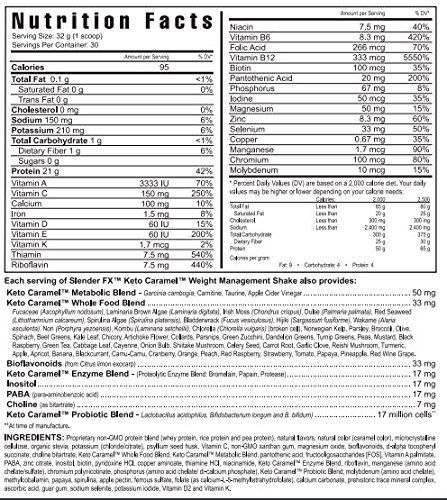This detailed close-up of the nutrition facts for the Slender FX Keto Caramel Weight Management Shake showcases essential nutritional information. The label specifies a serving size of 32 grams per scoop and notes that each container yields 30 servings. Clearly listed are the calorie count, total fat, cholesterol, sodium, potassium, total carbohydrates, and protein content. Additionally, the label provides a comprehensive list of included vitamins and their respective percentages per serving, ranging from niacin to molybdenum.

Prominently highlighted in bold print is the name of the product, "Slender FX Keto Caramel," along with detailed descriptions of its proprietary blends: Keto Caramel Metabolic Blend, Keto Caramel Whole Food Blend, Bioflavonoids, Keto Caramel Enzyme Blend, PABA, Choline, Inositol, and Keto Caramel Probiotic Blend. While these key components are easy to read, other nutritional details are printed in lighter ink and smaller font, making them less legible. Despite this, the essential information about the product's ingredients remains accessible and detailed.